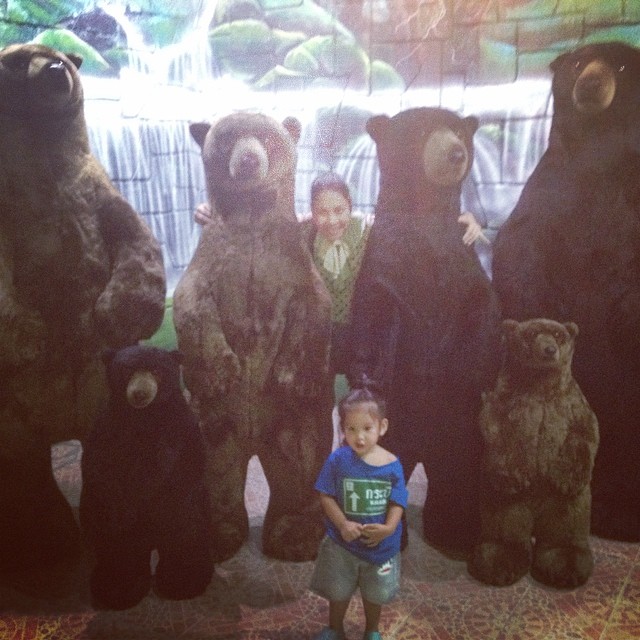In this photograph, an adult woman and a young toddler, likely her daughter, are posing with six large stuffed bears in front of a wall adorned with artwork depicting a waterfall cascading over rocks and surrounded by vegetation. The bears, arranged in a row and standing on their hind legs like humans, include four adults—two brown and two black—and two baby cubs—one brown and one black. The woman, dressed in a green top with black polka dots, stands between the two middle bears, draping her arms around them. The toddler, who appears about two years old, is positioned in front of the group. She has her hair up and is wearing a blue t-shirt and green shorts, though the image quality suggests it might also appear gray. The setting features a red and gold or burgundy and gold carpet. The detailed and colorful backdrop along with the variety of bear figures creates a visually engaging scene, even though the photograph is somewhat blurry and not of high resolution.